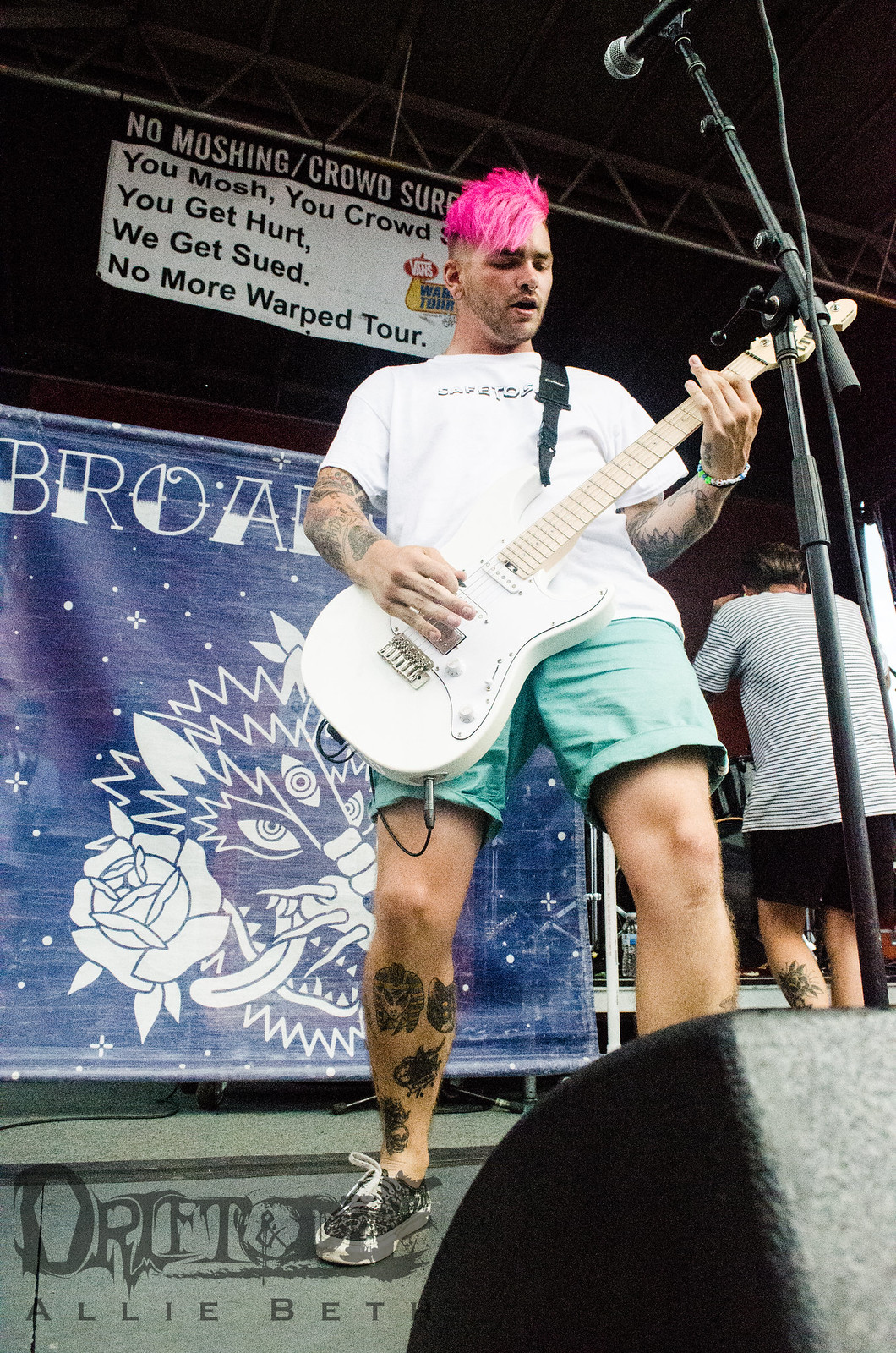This detailed photograph captures a captivating moment of a young musician, potentially a member of a punk band performing at the Vans Warped Tour. The artist, the focal point of the image, is a vibrant character with a distinctive bright pink tuft of hair, shaved close on the sides, and a slight stubbly beard. 

He's actively playing a white electric guitar, believed to be a Fender, his left hand expertly placed on the struts while his right hand strums with a pick. A black strap slung across his left shoulder helps support the guitar. He is dressed in a white short-sleeved t-shirt and mint green shorts, with black and white skate shoes. His arms and legs are heavily tattooed, contributing to his punk aesthetic. Leaning back from the hips, he appears to be mid-song, mouth open in expression. 

In front of him is a microphone on a black stand. The stage is situated outdoors under a black-roofed tent, with a large black speaker visible in the lower right foreground. Directly behind the musician is a striking blue banner adorned with the graphic of a white feline or lion’s head clutching a rose, partially obscured by the artist, and the readable text “B-R-O-A” suggesting the band name, potentially “Broadway.” 

Above this, a white banner with bold warnings about moshing and crowd surfing is prominently displayed, reading, "No moshing / crowd surfing. You mosh, you crowd surf, you get hurt, we get sued, no more Warped Tour.” This banner slightly obscures part of the stage’s metal overhead structure. Further in the background to the right, partially hidden, stands another person facing away from the camera, dressed in a white jacket and black shorts, further adding to the depth of the scene. 

This dynamic composition encapsulates the energy and environment of live punk rock performance.